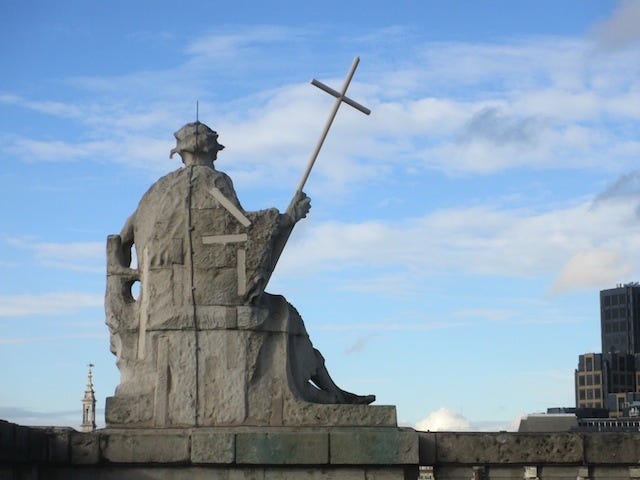This image showcases a large stone statue of a robed man seated on a tall, dark gray concrete wall, with his back facing the camera. The statue, which features a head covering and detailed armrests on the chair, holds a tall, thin white cross in its right hand. The scene is set against a pale blue sky with white and some darker, overcast clouds. Below and to the right of the statue, the tops of skyscrapers are visible, while to the left, the distinct outline of a small church tower peaks over the bottom edge of the wall. The overall palette consists of varying shades of gray and concrete, harmonizing with the subdued and serene atmosphere of the scene.